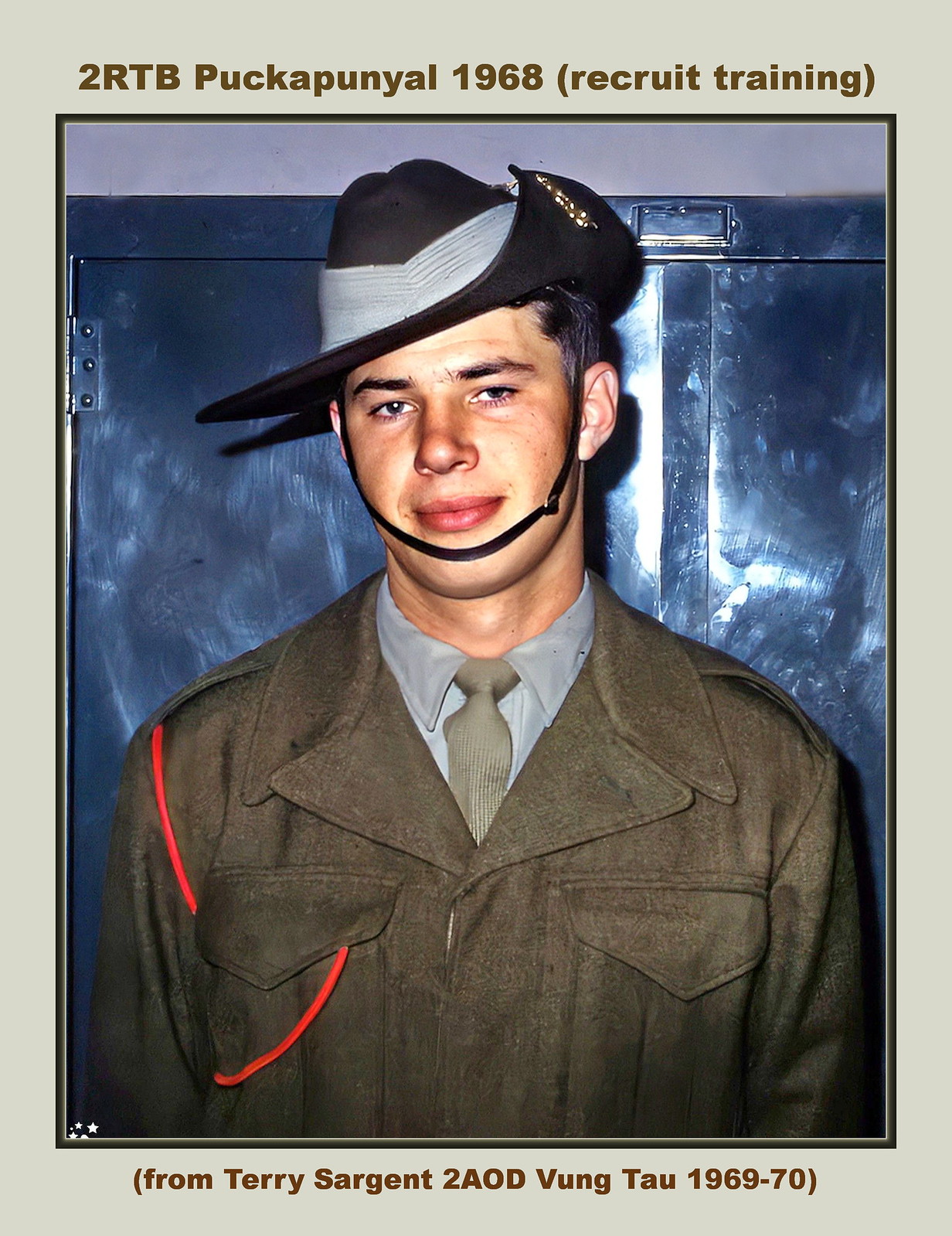The tall rectangular image features a photograph bordered by a light greenish-gray digital frame, which is wider at the top and bottom than on the sides, with a dark green-gray inner border. At the top, in bold brown font, the text reads "2RTB Puka Punyal 1968 (Recruit Training)." At the bottom, in the same brown font, it reads "(From Terry Sergeant to AOD Vung Tau 1969-70)." The man in the photograph is smiling faintly and is shown from the chest up. He is wearing a light green collared shirt, a green tie, and a green jacket. The man's black fedora-shaped hat, which has a gray ribbon and a black strap, is situated above his chin. Behind him is a series of metal lockers.